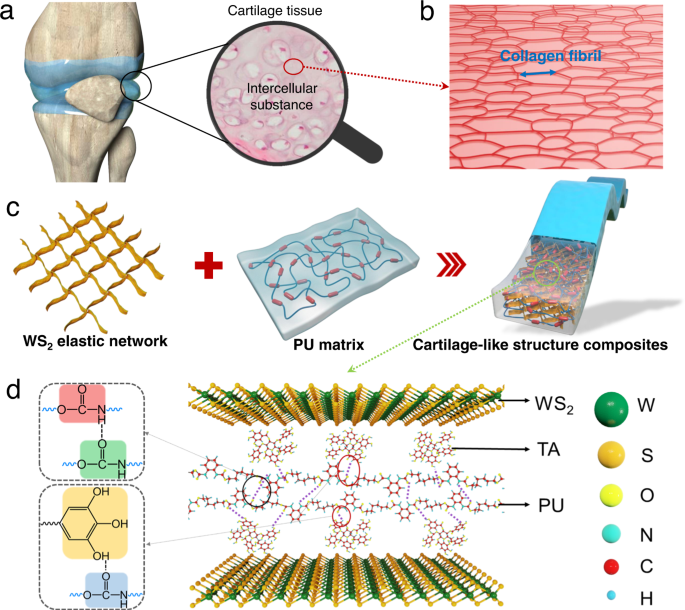This educational medical illustration, resembling a textbook diagram, comprehensively presents various interconnected scientific concepts. 

In the top left corner, labeled A, three bones converge at a joint, accompanied by a magnified view illustrating "intercellular substance". Just to the right at the top, labeled B, is a red cellular depiction indicating a "collagen fibril". In the top center-left, labeled C, the image features a "WS₂ elastic network" paired with a "PU matrix", connected to a blue wavy structure indicative of "cartilage-like structure composites".

At the bottom left, labeled D, is a chemical diagram containing two molecular representations within colored squares. In the bottom center, a larger, unlabeled molecular series features items like WS₂, TA, and PU to its right. Finally, on the bottom right, a sequence of decreasingly sized balls are color-coded and labeled: a large green sphere marked W, followed by smaller yellow spheres labeled S and O, an aqua ball labeled N, a small red ball labeled C, and the tiniest blue ball labeled H.

The image systematically organizes these scientific elements with clear labels and arrows, aiding in the educational depiction of cartilage tissue, collagen structures, and molecular compositions.